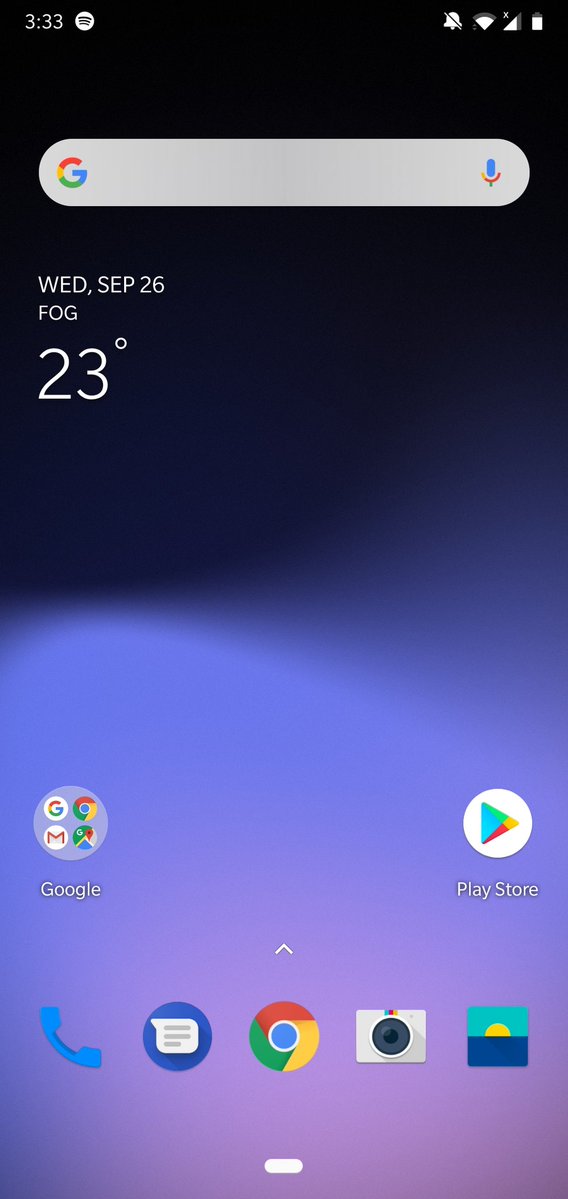The image displays a cell phone home screen featuring a color gradient background. The gradient transitions from an almost black color at the top, to a darker bluish-purple, then into a bright bluish-purple in the middle, and finally into a vibrant purple at the bottom. At the top of the screen, the time is shown as "3:33" AM/PM, accompanied by a white Spotify logo to its right. In the upper right-hand corner, there are various status indicators, including a muted notifications bell, data and Wi-Fi signal indicators, and a nearly full battery icon.

Below the time, there's a Google search bar with the Google "G" logo on the left and a microphone icon on the right. The search bar is empty, indicating no current text. Beneath the search bar, the date is displayed as "Wednesday, SEP 26," with a weather update showing "fog" and a temperature of "23 degrees."

Lower down on the home screen are several app icons arranged in a grid-like formation. These include icons for Google, the Play Store, Phone, Messages, Google Chrome, a Camera or Photos app, and a weather app featuring a sunrise icon.